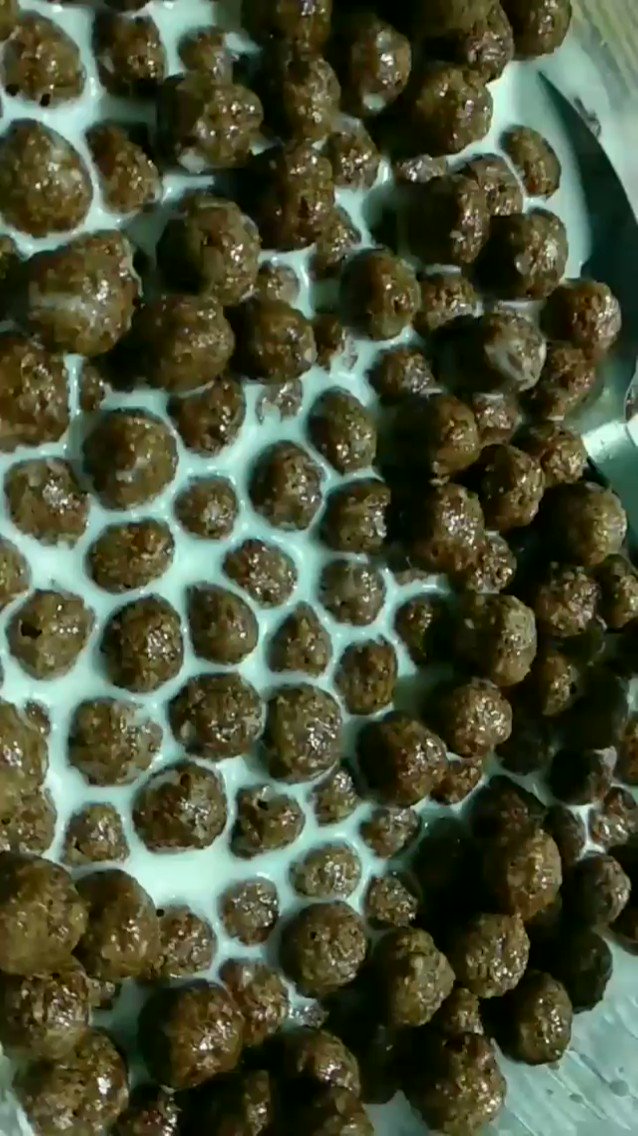This image is a close-up of a bowl of chocolate breakfast cereal, specifically resembling cocoa puffs or cocoa pellets. The cereal, which consists of little dark brown balls, is floating in white milk, giving the appearance of volcanic rocks mingling in liquid. To the right side of the image, a silver spoon is positioned, poised to scoop up a spoonful. The picture is vertically oriented and somewhat blurred, with a tight, narrow crop that predominantly frames the cereal and milk. The photograph, seemingly taken with a camera and perhaps tilted sideways, suggests the bowl is placed on a grayish to white distressed wooden table, with speckled dots adding texture to the surface. The background detail is minimal, allowing the focus to remain on the symmetrically sized chocolate cereal pieces. No text, date stamp, or artist signature is visible in this rectangular, quality-compromised image.